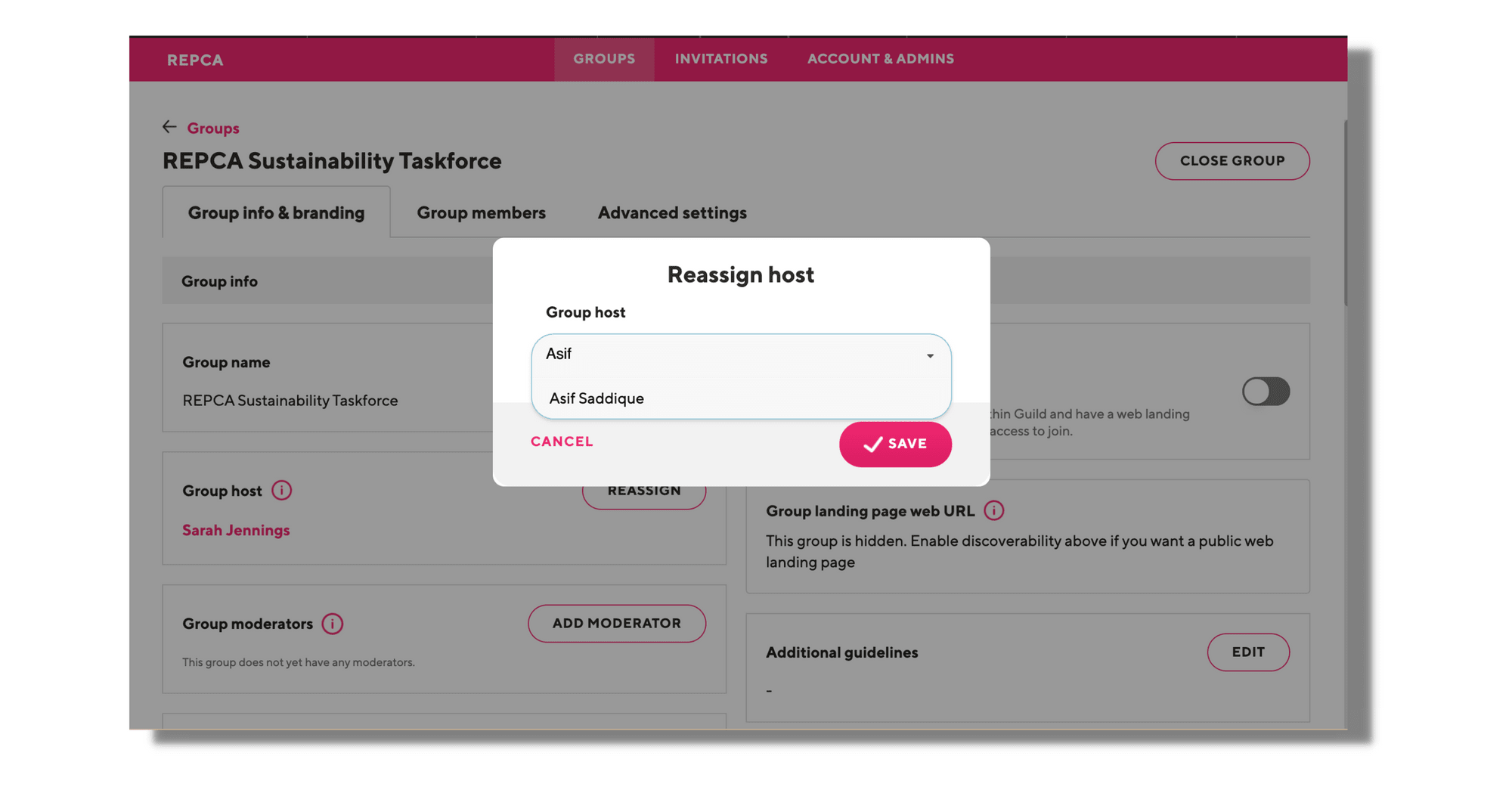The image depicts a section of a website interface focused on group management within a platform called REPCA. At the very top, a burgundy border displays navigation options in gray lettering: "Groups," "Invitations," "Accounts," and "Admins." Below this border, the background turns gray, and a left-pointing arrow accompanies the word "Groups."

Within this section, we see the title "REPCA Sustainability Task Force" prominently displayed. On the right side next to the title, a button labeled "Close Group" is visible. Beneath the main title, there are tabs for "Group Info and Branding," "Group Members," and "Advanced Settings." The current view is on the "Group Info" section.

In this "Group Info" section, there are entry designations for "Group Name," "Group Host," and "Group Moderators." Notably, the "Group Host" entry is highlighted, indicating an attempt to change or reassign the host. Currently, the host is listed as Sarah Jennings. The "Reassign" tab has been clicked, prompting a white box to appear with the name "Asif Sadiq" inside. This indicates that the host name is in the process of being changed from Sarah Jennings to Asif Sadiq. At the bottom of this prompt, options to "Cancel" or "Save" the changes are available.